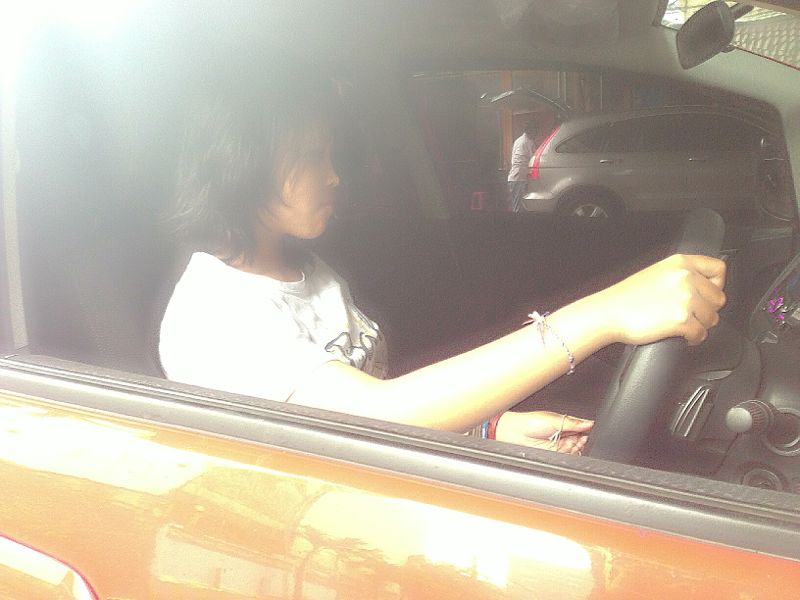The image features an Asian woman with brown skin and short, straight, dark hair, seated in the driver's seat of a car. She wears a white shirt with black letters "BA" on it, and her hair reaches down to the collar of the shirt. Her right hand, adorned with a purple and white bracelet, rests on the top of the black, rounded steering wheel, while her left hand, which sports three to four bracelets in red, blue, and brown, is positioned near the bottom of the wheel. The woman's focused gaze is directed forward, captured in a slightly blurry photograph with a lot of light coming in from the top left of the image.

The car's interior features a black dashboard and door trim, with some purple accents visible in the dashboard area. The door panel, door handle, and a portion of the car's exterior have a glossy orange finish that reflects the street scene outside. The car's window is rolled down, allowing a clear view of the surroundings.

In the background, through the car window, there's a silver vehicle, possibly a minivan or SUV, with the back trunk open. A man, wearing a white shirt and gray pants, stands at the rear of the silver vehicle, looking into the trunk. Beyond him, a grayish-white building with orange elements can be seen through the first car's windshield. The scene is well-lit, suggesting that the photograph was taken in daylight.